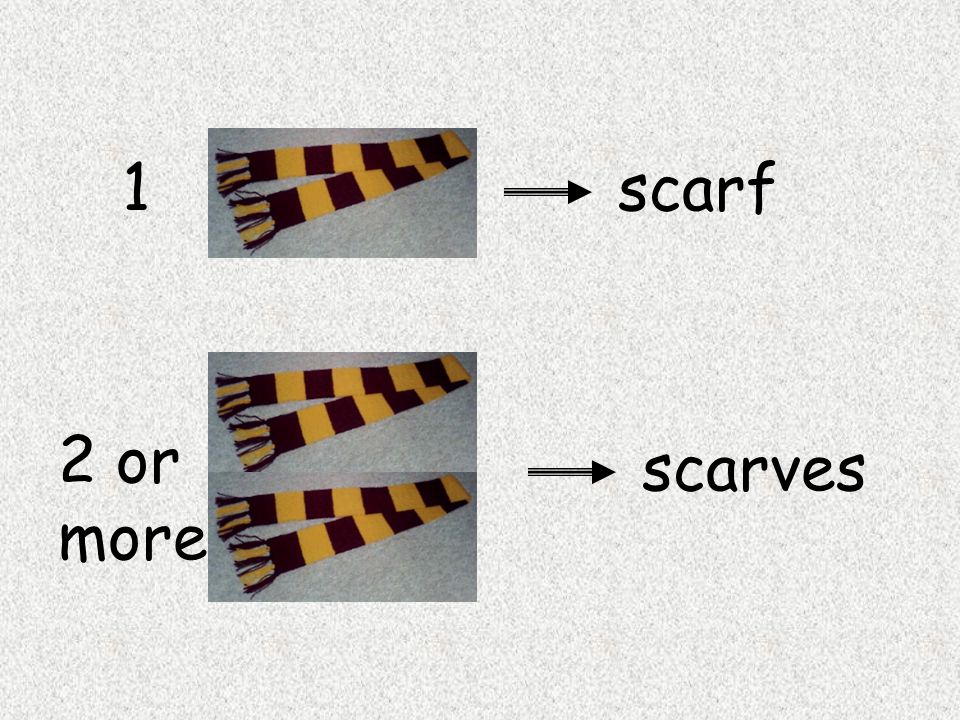In this image, which appears to be part of a PowerPoint presentation teaching the concept of singular and plural, there is a textured grayish-blue background. The image is divided into two main sections. The top section displays a single maroon and yellow scarf, which features alternating boxes in these colors along with matching tassels. To the left of this scarf, the text reads "one," and an arrow points to the word "scarf" in black text on the right.

The bottom section mirrors the first but shows two scarves of the same maroon and yellow pattern. To the left, the text reads "two or more," and an arrow points to the word "scarves." This section aims to illustrate the difference between the singular "scarf" and the plural "scarves" (noting the change from 'f' to 'ves').

The repeated maroon and yellow colors are reminiscent of the University of Minnesota's color scheme, helping to visualize the design of the scarves. The overall presentation style clearly aims at educational purposes, particularly to explain the pluralization of nouns.